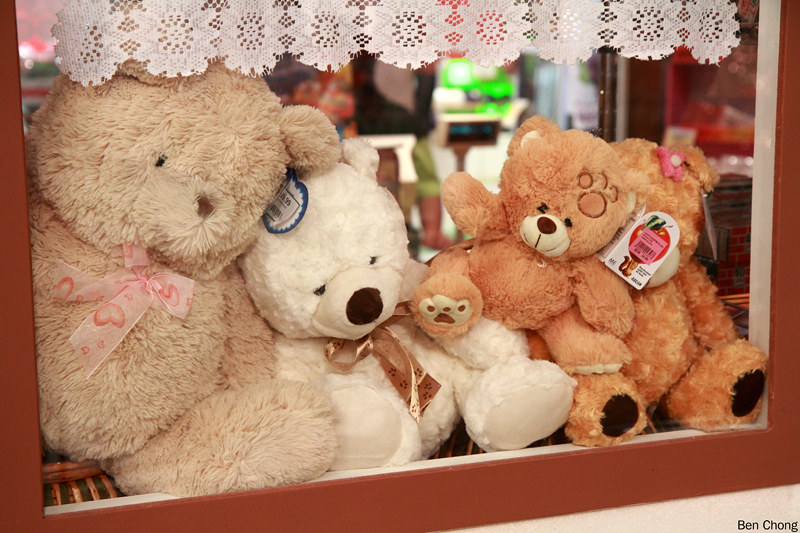The photograph captures a display of four teddy bears arranged upright against each other behind a pane of glass, framed by a red-painted wooden structure designed to resemble a window, complete with a hanging lace curtain. On the far left, there's a light brown bear adorned with a pink bow. Next to it, sits a white teddy bear with curly fur and a brown bow. The third bear in line is a caramel-colored bear featuring a sheer brown bow. Lastly, on the right is another caramel bear, distinguished by its black foot pads and a small pink hair bow. The background appears busy and blurred, suggesting the bears could either be part of a shop window display or potentially within a fairground grab machine, though the top of the setup is obscured, leaving their exact location ambiguous.